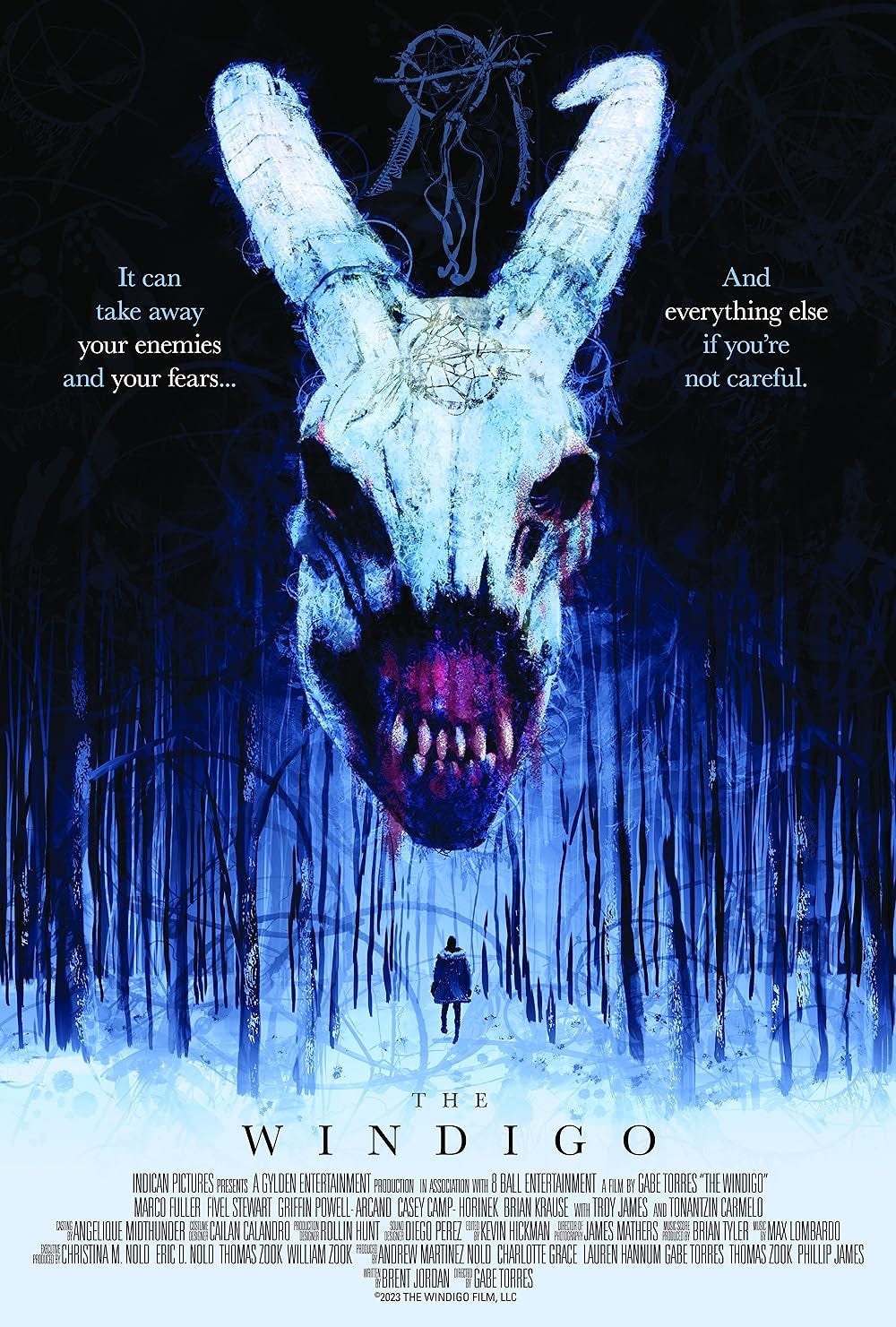The movie poster for "The Wendigo" prominently features a looming, partially skeletal deer skull with hollow eyes and exposed demonic teeth emerging from a broken nasal cavity, all rendered with a purplish hue. Goat-like horns curl out from the sides of the skull, but they are positioned more like deer antlers. Mysterious, magical inscriptions cover the skull, and an outline of a Native American dreamcatcher is visible above it. This ominous centerpiece hovers over a forested backdrop, painted in shades of blue, with a solitary figure clad in a fur-collared blue jacket walking into the woods. The tagline, "It can take away your enemies and your fears and everything else if you're not careful," arches near the horns. The poster's color palette includes bluish-white, red, black, and light bluish-purple hues, contributing to its eerie atmosphere. Credits at the bottom detail the film's production by Indykin Pictures, Glyden Entertainment, and 8 Ball Entertainment, directed by Gay Torres, marked as a 2023 release by The Wendigo Film, LLC.